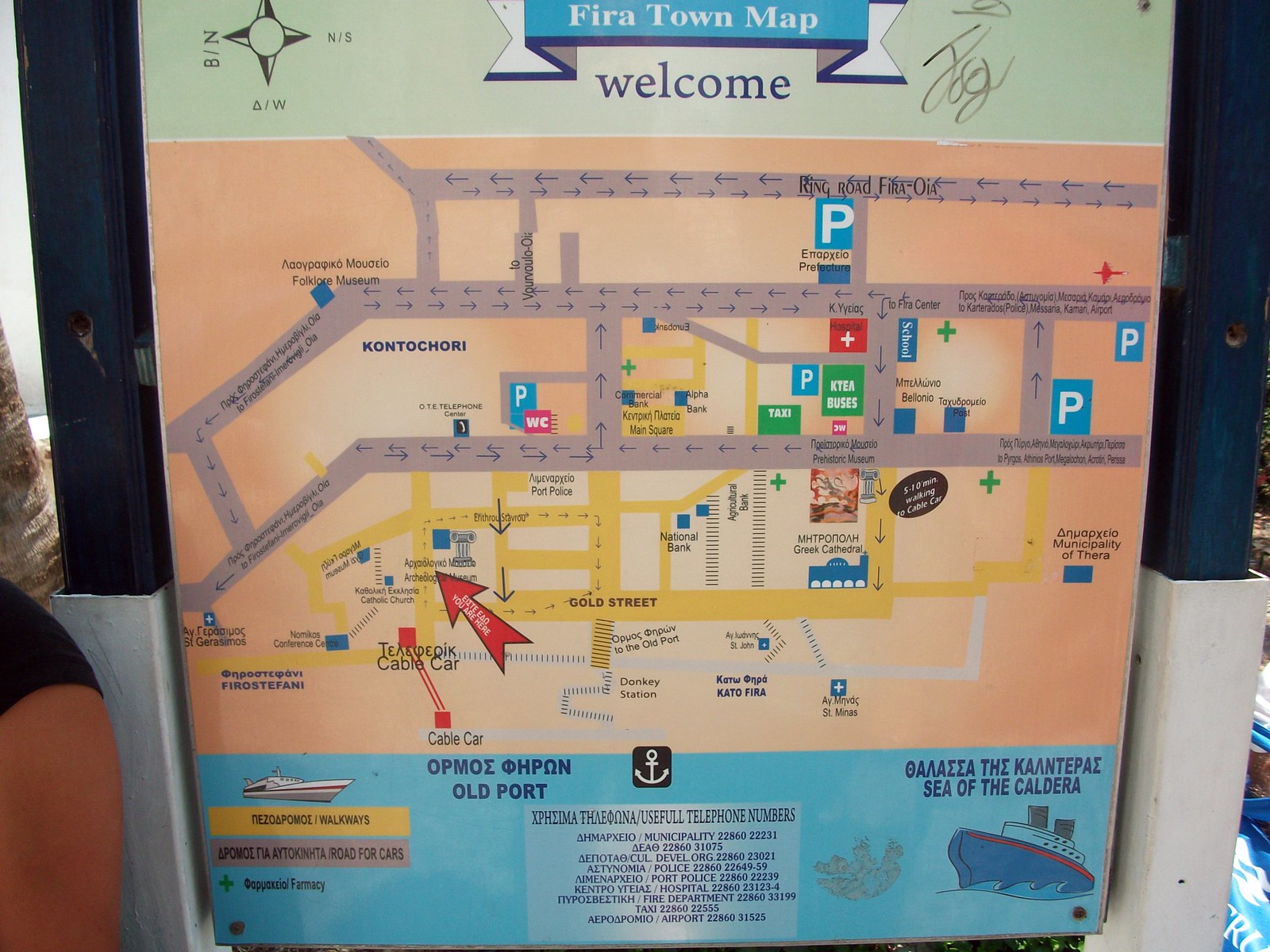This descriptive sign is likely found in a tourist area and features a detailed town map of Fira, Greece. The top of the sign bears a folded banner with the title "Fira Town Map" in white lettering against a light green backdrop, followed by the word "welcome" in blue on the green background. Adjacent to the welcome sign, on the left upper panel, there is a compass rose indicating the cardinal directions.

Beneath the header is the main town map, rendered in various colors including light orange, red, yellow, blue, white, black, green, and gray. This colorful schematic delineates roadways—some marked with arrows indicating directions—and parking lots symbolized by white "P" on blue squares. Additionally, essential services such as water closets (WC), a taxi stand, and KYEA buses are indicated by distinctive logos.

Among the notable landmarks on the map is Gold Street, highlighted in gold color. The map also identifies key locations like cathedrals and stores. The entire map section is set against a light brown backdrop.

Below the town map, there is a blue band stretching across the sign, featuring two intricately drawn ships. One ship, labeled "Sea of the Caldera," is a cruise ship named Gaia Thaikonthepak. The drawings and some inscriptions are presented in both Greek and English. Between the two ships' images lies a black background with a white anchor symbol. Directly below this section is a white panel displaying the telephone numbers of the sponsoring cruise ship company, alluding to their services in the area.

This sign effectively serves as a navigational and informational tool for tourists, providing a comprehensive overview of Fira's layout and essential services.